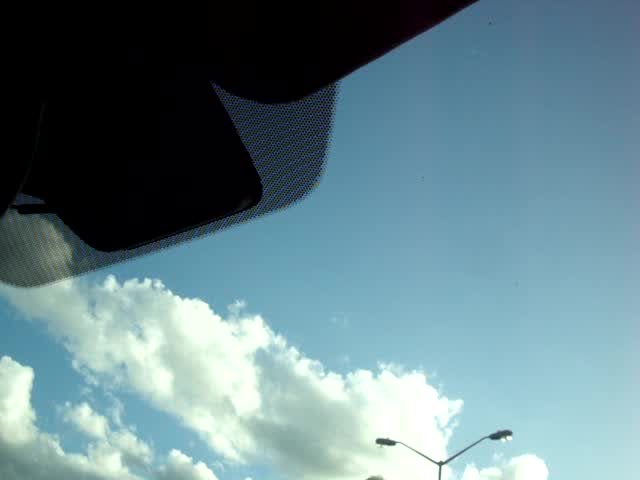The photo, taken from within a car, captures a unique upwards perspective. In the top left corner, the interior roof of the vehicle is visible, including the silhouette of a sun visor and a small, dimmable rearview mirror on the windshield. Just outside of the vehicle, the image showcases a street lamp with two fixtures branching out in a Y formation, standing tall against the sky. Above, the expansive sky dominates the scene, with most of it clear and blue. Towards the bottom of the shot, large, fluffy white clouds add a touch of contrast and texture to the otherwise pristine afternoon sky.